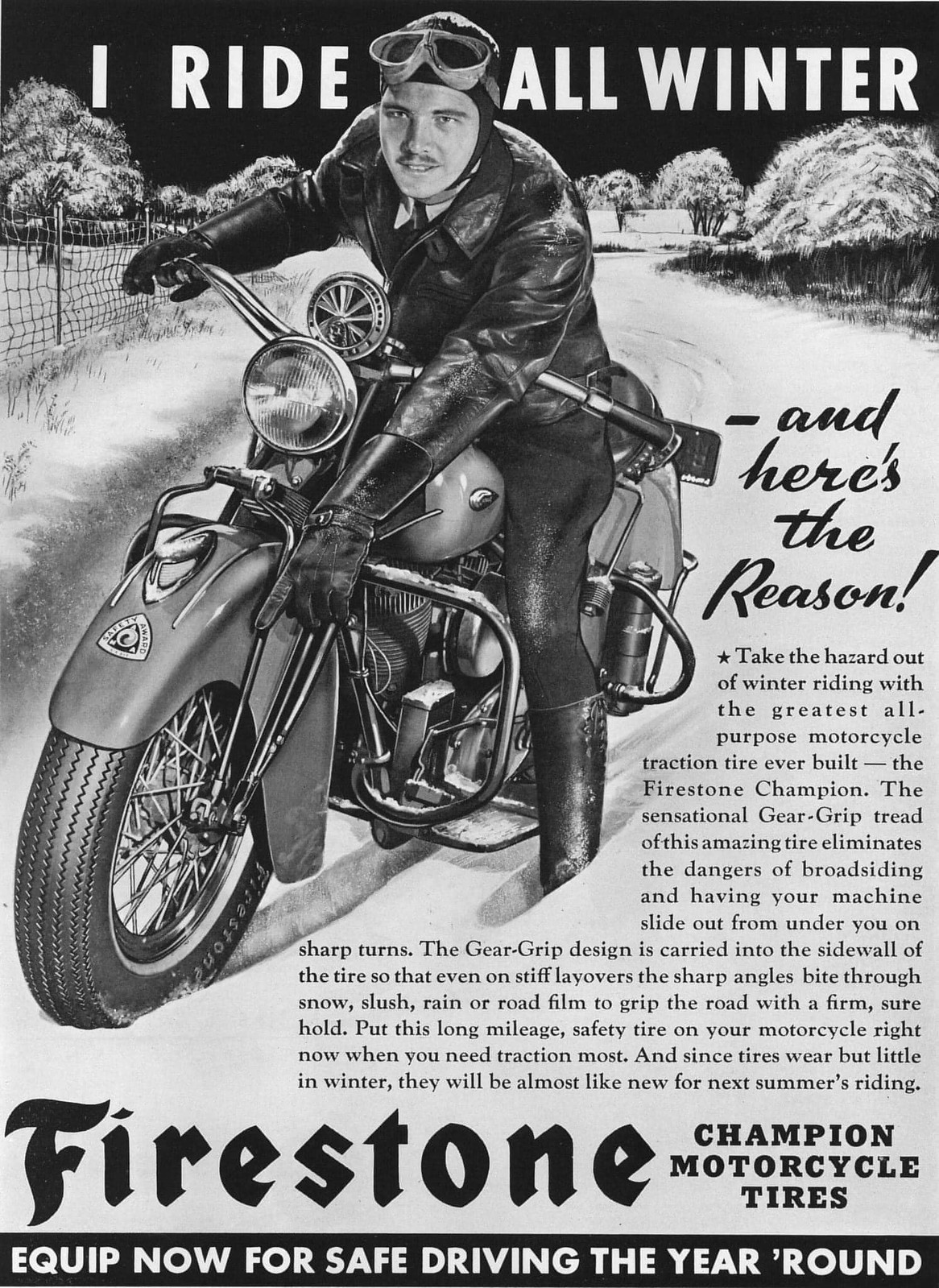This vintage black-and-white Firestone Tires advertisement highlights the exceptional performance of Firestone Champion motorcycle tires in winter conditions. Set against a snowy backdrop with trees covered in snow, the ad features a man riding a motorcycle equipped with these cutting-edge tires. The rider, dressed in a leather jacket, leather pants, dark gloves, and boots, also sports old-fashioned motorcycle goggles pushed up on his forehead. The bold white text at the top declares, "I ride all winter," followed by a detailed explanation: "Take the hazard out of winter riding with the greatest all-purpose motorcycle traction tire ever built, the Firestone Champion." The ad emphasizes the tire's sensational gear grip tread, designed to eliminate the dangers of broadside slides and sharp turns by biting through snow, slush, rain, or road film. The gear grip design extends to the tire’s sidewalls, ensuring firm traction even on stiff layovers. With the slogan "Equip now for safe driving the year-round" at the bottom, the ad encourages riders to install these long-mileage safety tires immediately for optimal traction during winter, guaranteeing they will remain almost like new for summer riding.